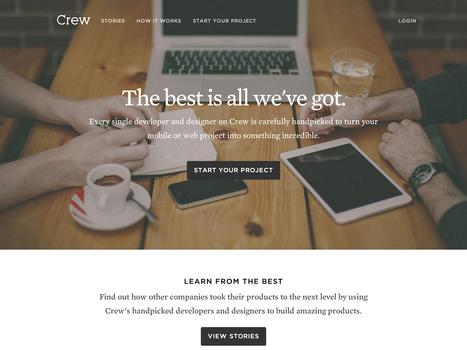The image is an advertisement for a group of programmers. At the top of the image, the company's name, "Crew," is displayed alongside three navigation links: "Stories," "How It Works," and "Start Your Project." These elements are superimposed on a background image of a pine board table. 

On the table sits a laptop, positioned in the middle and facing the viewer, although it appears unused. Two individuals are present in the image; one is writing in a paper notebook while drinking a beverage that looks like an espresso, and the other has a glass of water and a small tablet, which he is not currently using. Although you cannot see their faces, their arms extend into the frame, adding a human touch to the scene. The person with the tablet is wearing a watch with a black face, silver body, and black armband.

Centered text on the image states, "The best is all we've got. Every single developer and designer on Crew is carefully handpicked to turn your mobile or web project into something incredible." Below this text is a black button labeled "Start Your Project."

Below the image, against a white background, there is additional text that reads, "Learn from the best. Find out how other companies took their products to the next level by using Crew's handpicked developers and designers to build amazing products." Following this, a "View Stories" link is provided, inviting users to explore further.